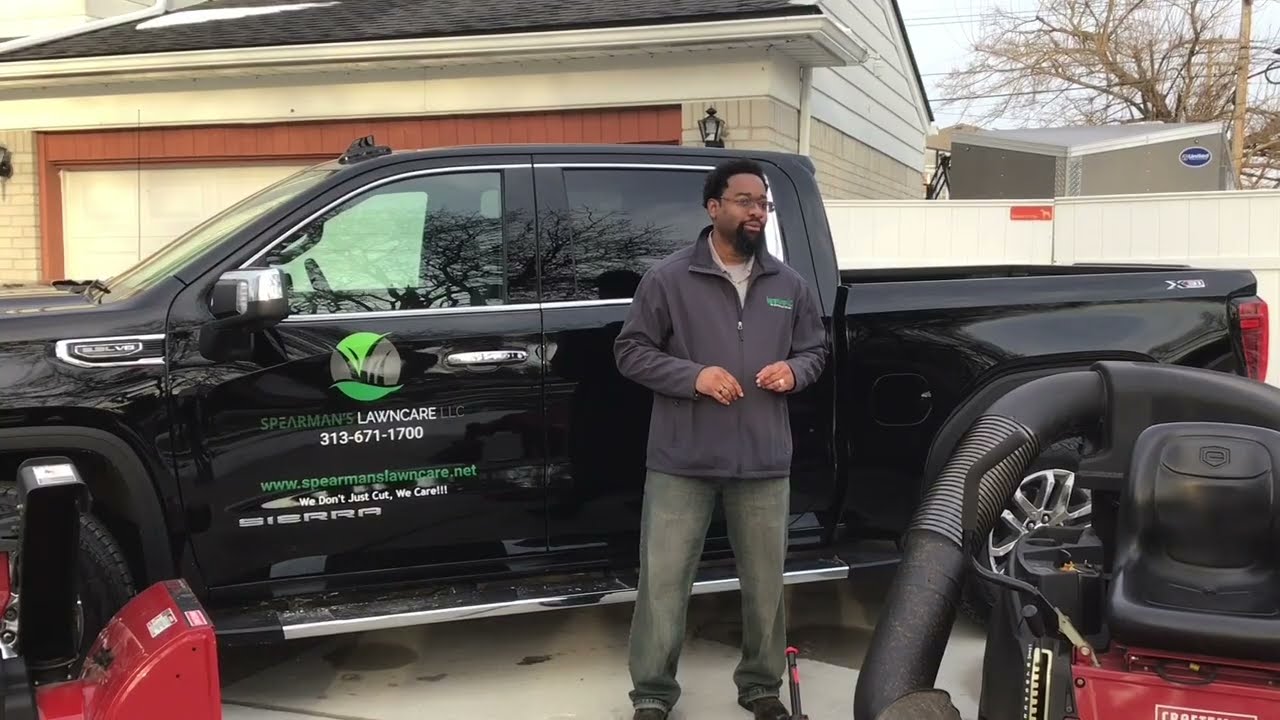A detailed photo depicts an African-American man standing beside a glossy black GMC Sierra Dually pickup truck adorned with extensive chrome detailing, including door handles, extended side mirrors, step sides, and window trim. The truck features the logo "Spearman's Lawn Care, LLC" and the phone number "313-671-1700" prominently displayed on the driver's side door. The man, middle-aged with black hair, a black goatee, glasses, and wearing a blue or gray fleece with a logo on the left chest, stands confidently beside the crew cab. He is dressed in jeans and possibly a wedding ring. The scene is set in what appears to be a middle-class neighborhood driveway, near a garage, with visible elements such as a grass mower, typical lawn care equipment, and potentially a lawn care worker attending to machinery nearby. The backdrop includes a white garage with a brown and white door, a fence, and overhead wires, contributing to the suburban setting.